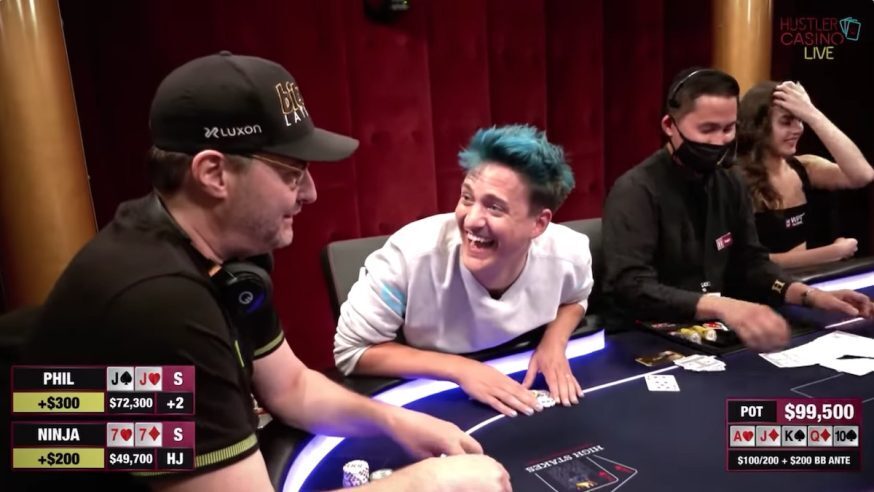The image captures a lively moment from a professional poker game. The four players surround a blue neon-lit poker table with a plush red velvet backdrop adorned with shiny gold posts. On the far right, a young Caucasian woman in a black tank top and belly shirt, hand on her head and laughing, sits beside an Asian man with his hair pulled back and a black face mask. The Asian man, acting as the dealer, is wearing a black shirt and black earphones with a microphone. Next to him, a man in a white long-sleeved shirt, with the tips of his hair dyed blue, is bent over laughing. Completing the scene, at the table's end, is a man wearing glasses, a brown cap, and headphones around his neck.

The bottom left of the image displays the names and current standings of the players: Phil is up $300 with a pair of jacks, and Ninja is up $200 with a pair of sevens. A pot of $99,500 is indicated in white text against a black background. The table shows an ace, jack, king, queen, and ten, indicating that Phil is likely to win. A "Casino Live" graphic is positioned in the top right corner, underscoring the professional and dynamic atmosphere of the game.